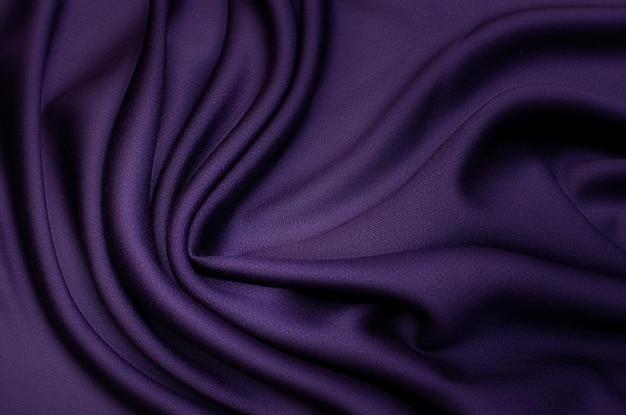The image is a horizontally rectangular photo featuring a deep purple piece of cloth. This fabric appears to be soft and smooth, resembling satin or silk, and has a subtle, almost shiny quality. It is not laid out flat but rather features natural folds and swirls, especially noticeable running from the top left down to the bottom right. The varying shades of purple, from dark to light, are due to the way light and shadows interact with the fabric's texture. There is no border, background, text, people, or any other elements in the image, the focus entirely on the richly colored and somewhat glossy material, possibly resembling a folded tablecloth, sheet, or blouse.